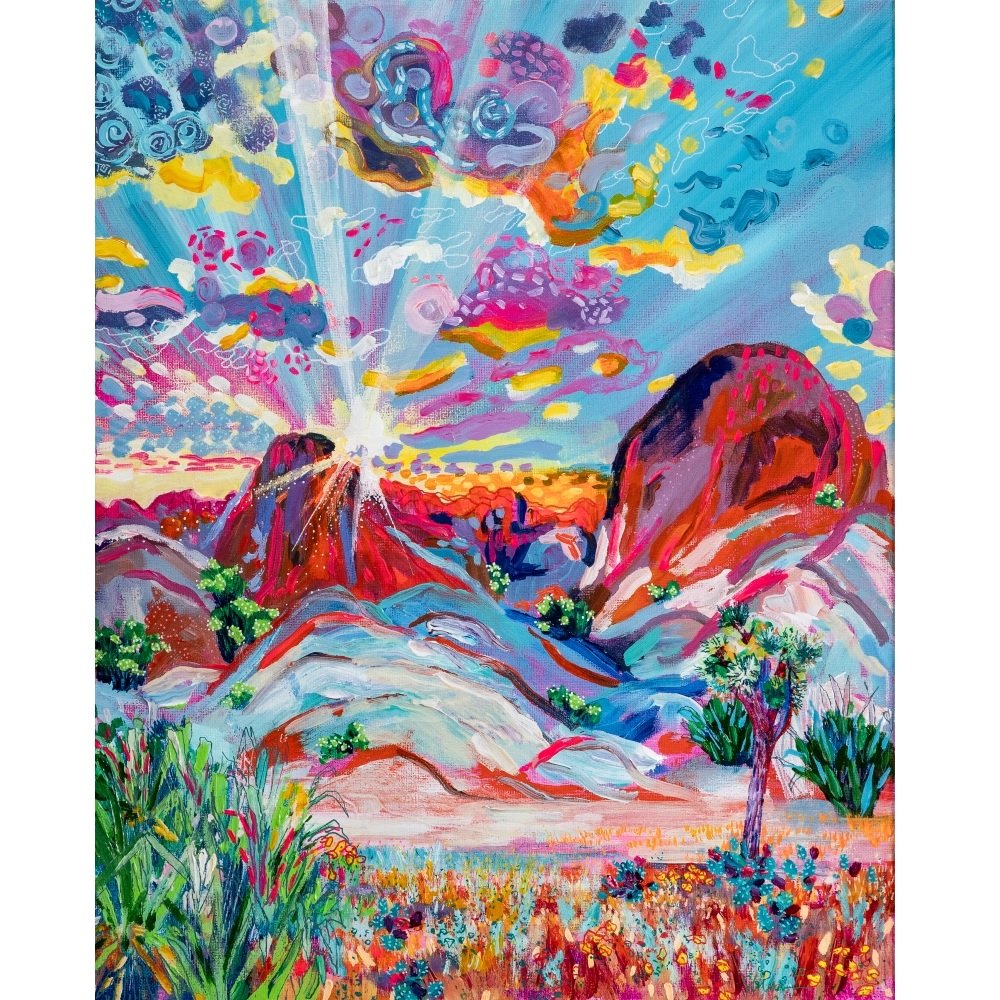The painting is an explosion of vibrant colors and abstract designs depicting a natural landscape. The upper portion of the artwork features a dynamic sky filled with swirling patterns and circles in shades of purple, blue, yellow, pink, and white. A brilliant white sun is nestled behind an array of mountains, casting light-colored rays that blend seamlessly with the whimsical sky. The mountains themselves are a patchwork of browns, blues, pinks, grays, and whites, with lighter areas that could represent snow or simply artistic light accents.

In the midground, sparse trees and bushes sprout from the rocky terrain, their foliage an eclectic mix of yellow, blue, pink, brown, green, and white hues. The lower portion of the painting transitions into a diverse foreground, highlighting a dirt area surrounded by an abundant variety of vegetation painted in the same vivid palette. The result is an intricate and colorful abstract landscape where each element, though stylized, is distinctly recognizable and harmoniously blended into the composition.